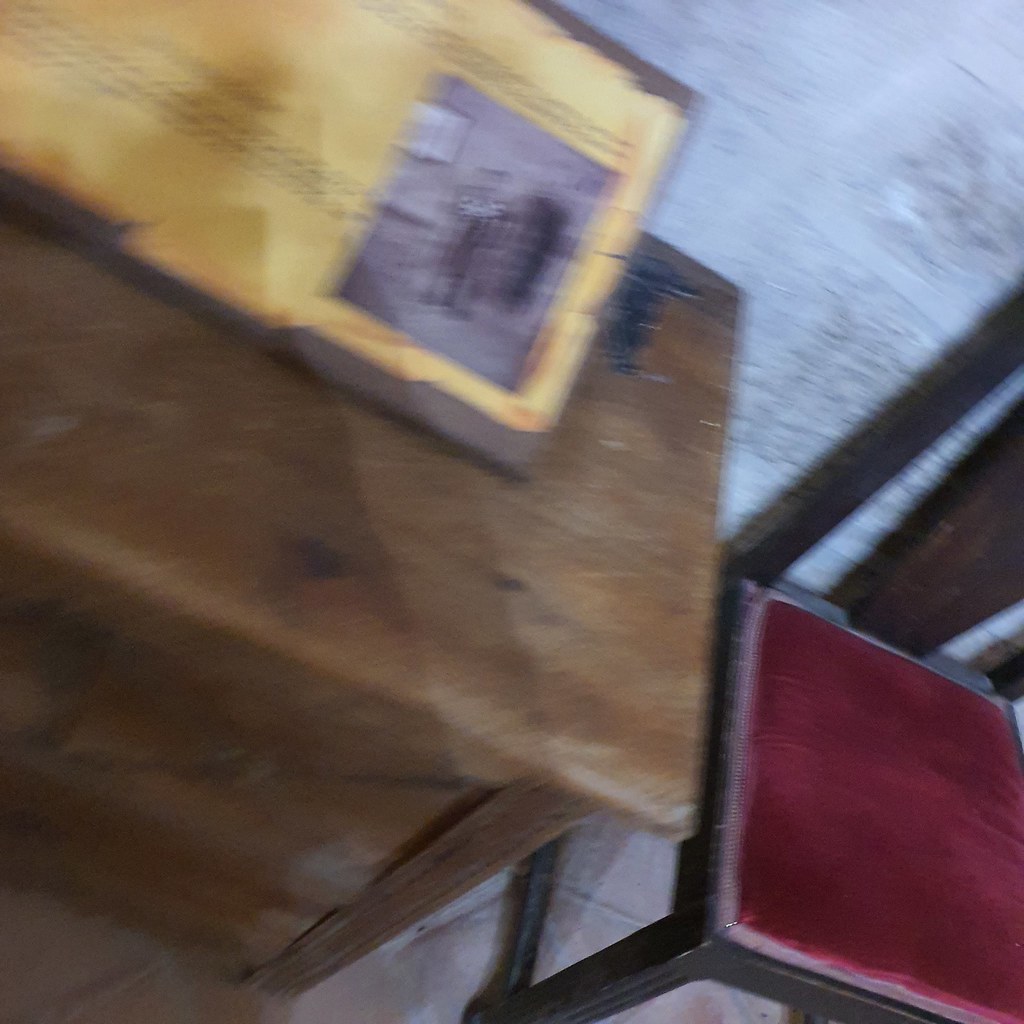The photo captures a scene featuring several objects, though it is somewhat out of focus. In the center of the image stands a brown wooden stool, designed with four sturdy legs and topped with a square, red velvet cushion. The cushion is bordered by a lighter shade of red fabric, delineating its edges. Adjacent to the stool is a brown wooden storage container, adorned with black hinges, giving it an antique appearance. Despite the blurred quality of the image, a yellow and brown rectangular object can be discerned perched on top of the storage container.